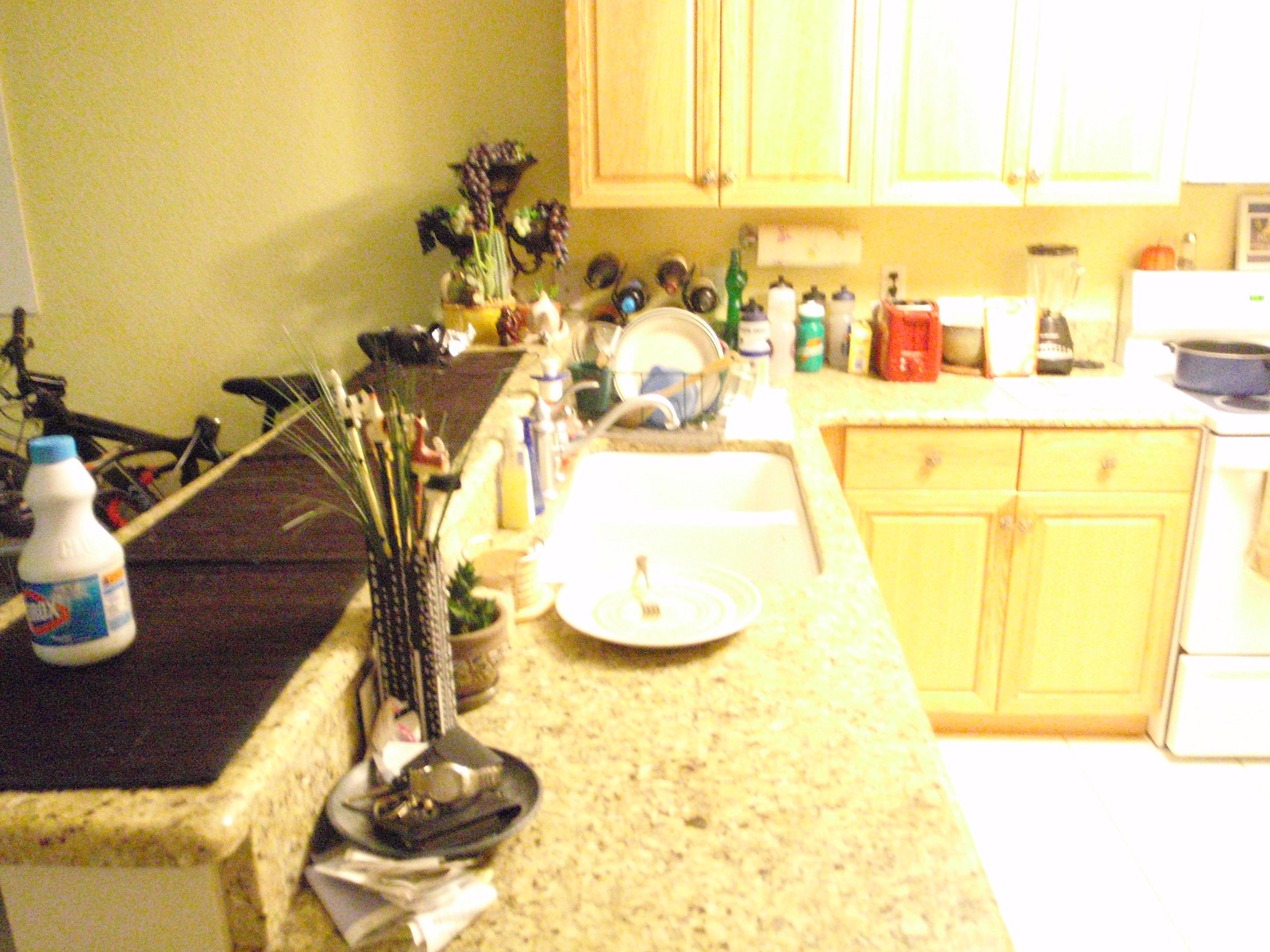In the image, we see a cozy, compact kitchen likely situated within an apartment. The left side of the kitchen features a granite countertop, subtly tinged in light yellow, bearing a bottle of Clorox bleach. Moving right, near the sink, several dishes are laid out to dry, with a solitary dirty dish placed on the counter to the left of the sink. 

The back counter houses an organized yet bustling array of items. Adjacent to the stove, there are multiple water bottles, a toaster, a blender, and a neat rack containing several wine bottles. The backdrop of this scene is a light yellow wall, complementing the light wood material of the overhead cabinets, whose natural grain contributes to their yellowish appearance.

This setting is bathed in the warm hue of light yellow, which dominates the color palette of the photograph, lending a cozy and welcoming atmosphere to the small kitchen space.